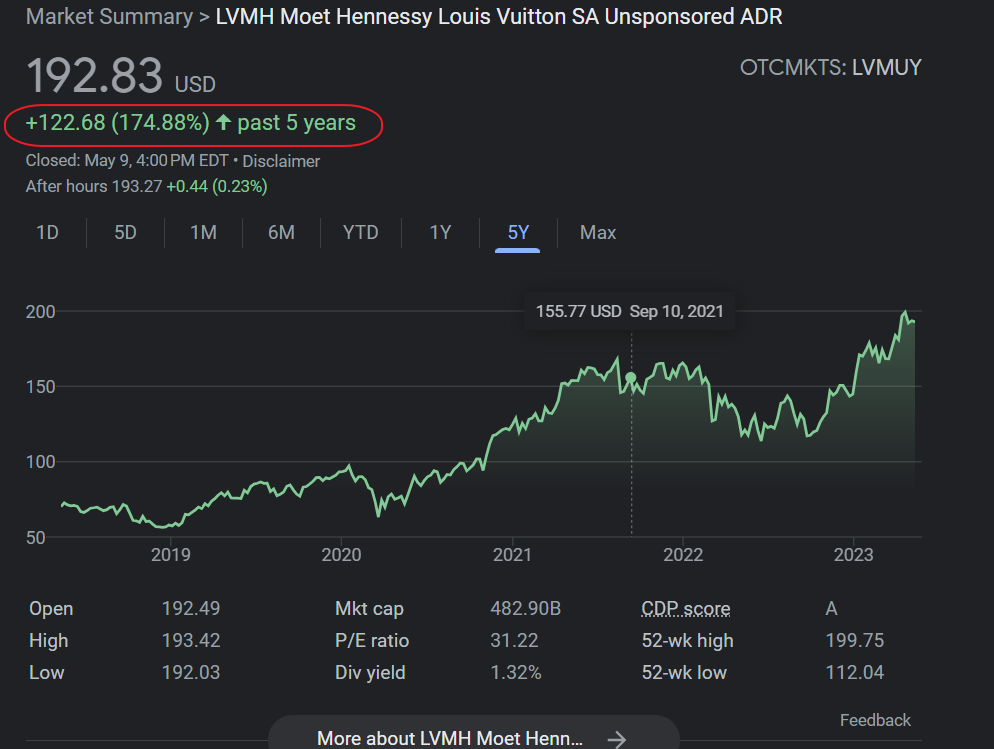Market Summary for LVMH Moët Hennessy Louis Vuitton, Unsponsored ADR (LVMUY):
- Current Price: $192.83 per share (USD)
- Performance: Highlighted in red is a green text showing an increase of $122.68, which represents a 174.88% growth over the past five years.
- Data Closing Time: Closed on May 19th, 4 p.m. Eastern Daylight Time.

Below the summary, a five-year stock performance graph is displayed, indicating significant price movements, including a notable price of $155.77 on September 10th, 2021. 

Key Metrics:
- Open Price
- Daily High/Low
- Market Capitalization
- Price-Earnings (P.E.) Ratio
- Dividend Yield
- CDP Score
- 52-Week High/Low

The chart features a black background with green graphical elements, providing a visually concise summary of the stock's performance.